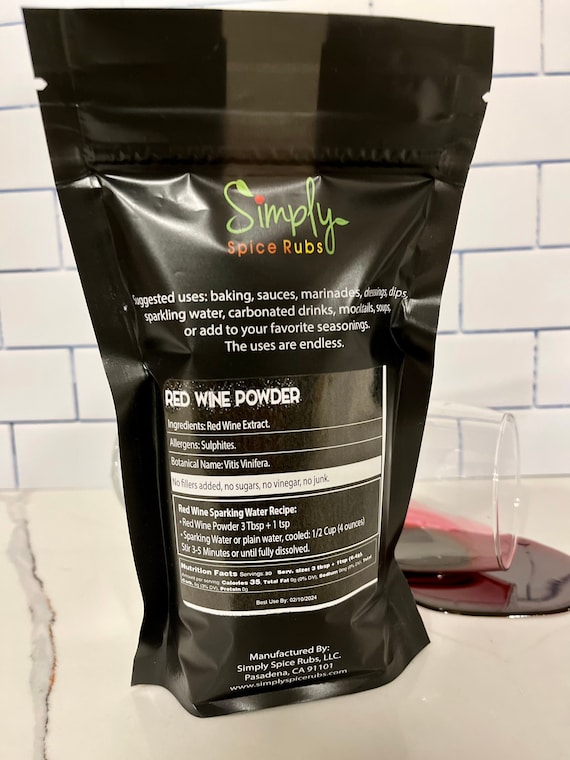The vertical color photograph captures a sleek, black resealable pouch from Simply Spice Rubs, prominently displaying the bold white and multicolored text. The front of the pouch features a large transparent window through which the vibrant red wine powder can be seen. The elegant text on the bag describes the versatile uses of the red wine powder, including baking, sauces, marinades, dressings, dips, sparkling water, carbonated drinks, mocktails, soups, or as an enhancement to favorite seasonings. The ingredients list highlights red wine extract, specifying allergens such as sulfites, with assurances of no fillers, sugars, or vinegar. A recipe for red wine sparkling water is included at the bottom. The text also notes the product's botanical name, "Vitis vinifera," and its origin from Simply Spice Rubs LLC, based in Pasadena, California. The image situates the pouch on a marbled white countertop against a white subway tile background, with a vibrant visual of a spilled glass of red wine, adding a touch of drama to the composition.